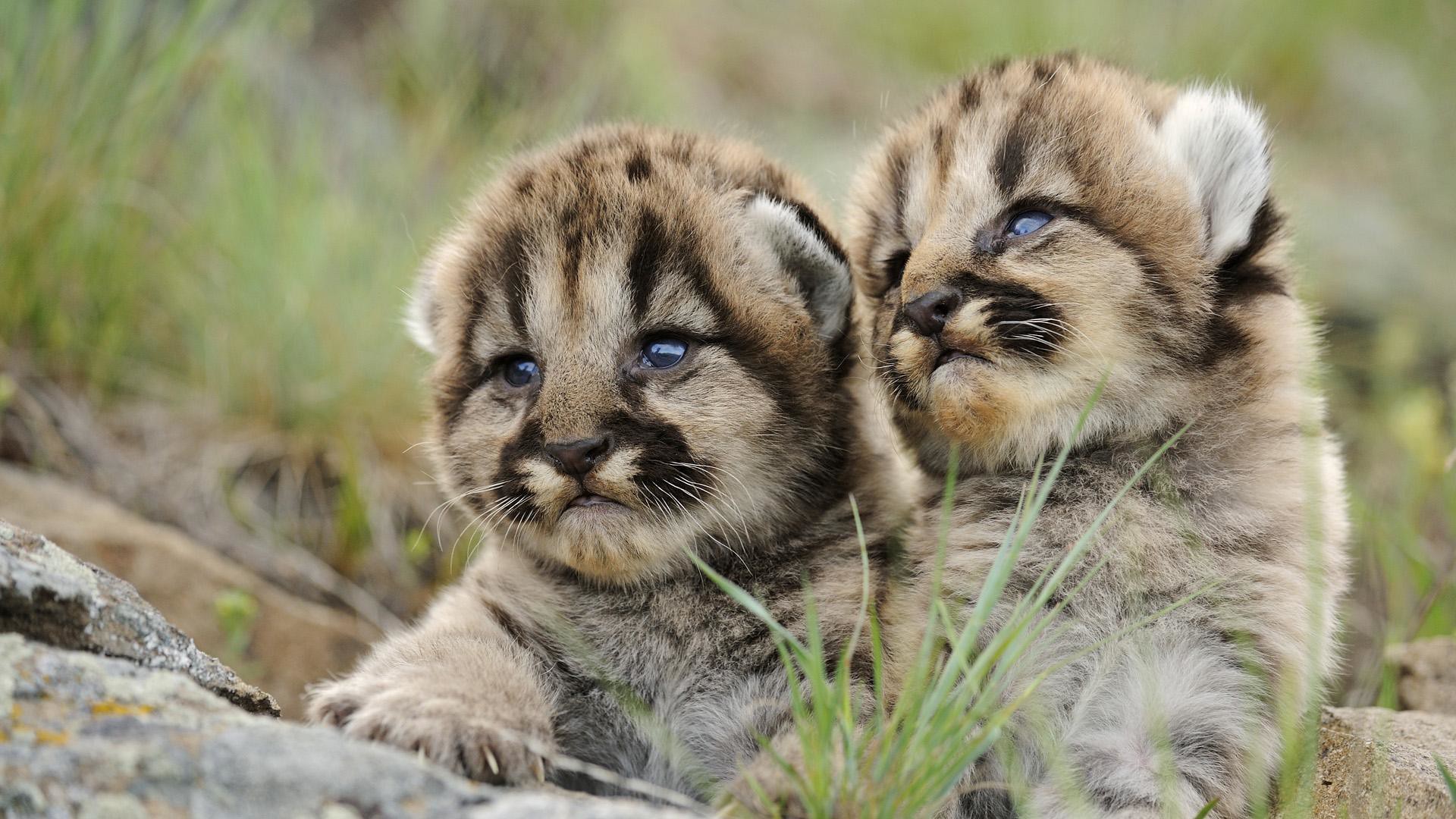The image features two young wildcat cubs, possibly bobcats or lynxes, nestled close together on a rocky terrain surrounded by patches of wild grass. The cubs exhibit a distinctive fur pattern, predominantly tan, dark brown, white, and grey, with noticeable stripes on their faces and the tops of their heads. This pattern includes intriguing markings around their eyes, forming an 'M' shape on their foreheads, and white specks on their cheeks. Both cubs have striking dark blue eyes and large paws with visible talons. The background, blurry and out of focus, further accentuates their clear and crisp figures, emphasizing the juxtaposition of the green weeds and the rocky ground in this natural setting.